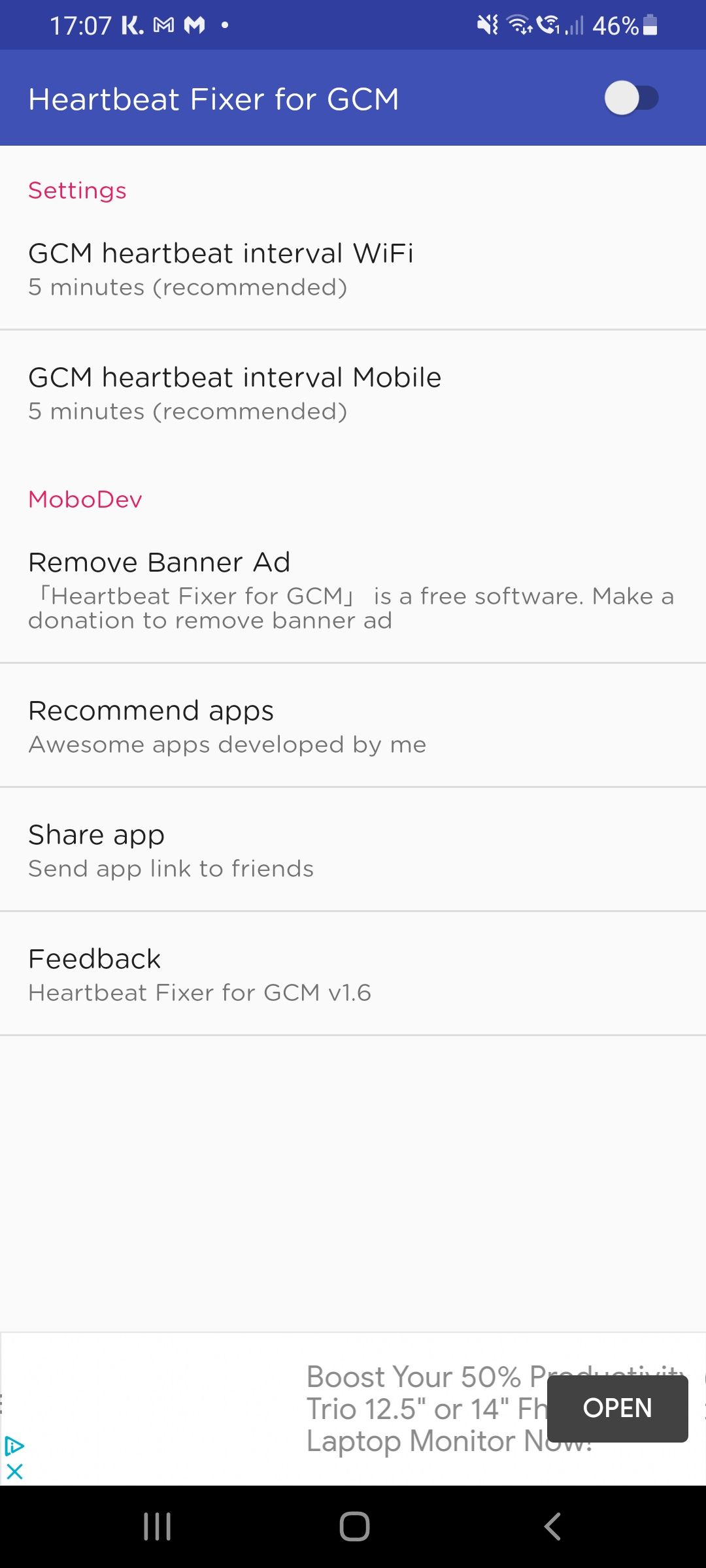A smartphone screen displays a webpage with a mixture of functional settings and promotional content. The time displayed in military format reads 17:07, translating to 5:07 PM. The phone's battery is at 46% power. The main feature highlighted is "Heartbeat Fixer for GCM," which can be toggled on or off. 

Under the main feature, several settings are listed: "GCM Heartbeat Interval, Wi-Fi," set to a recommended 5-minute interval, and "GCM Heartbeat Interval, Mobile," also set to a recommended 5 minutes. Both settings are written in a grayish-black text.

A section labeled "Mobo Development" appears in red, followed by an option to "Remove Banner Ad" which notes that "Heartbeat Fixer for GCM J is a free software." Users are invited to make a donation to remove the banner ad. 

Additional sections include "Recommended Apps," and "Awesome Apps Developed by Me," along with a "Share App" function to send the app link to friends. For feedback, the app version is listed as "Heartbeat Fixer for GCM Volume 1.6," with a claim of boosting productivity by 50%. Finally, there's a button with a prompt to "Open in Your Laptop Monitor Now."

The webpage design features a mix of colored text with critical settings in red and informational text in grayish-black.